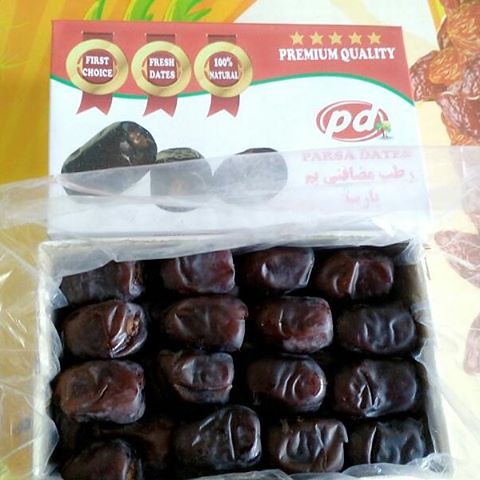The image shows a top-down view of an open package containing dried dates, organized neatly in four rows of four dates each, with an additional layer of dates beneath. The dates are encased in clear plastic. The lid, positioned just above the box, is predominantly orange and white and features prominently in the composition. It bears elaborate gold ribbons that highlight phrases such as "First Choice," "Fresh Dates," and "100% Natural." The packaging also boasts a "Premium Quality" label with five gold stars adorning the top right corner. Near the bottom of the package, the logo "PD," likely representing "Parsa Dates," appears along with additional wording, possibly in Arabic, amplifying the product’s authenticity.